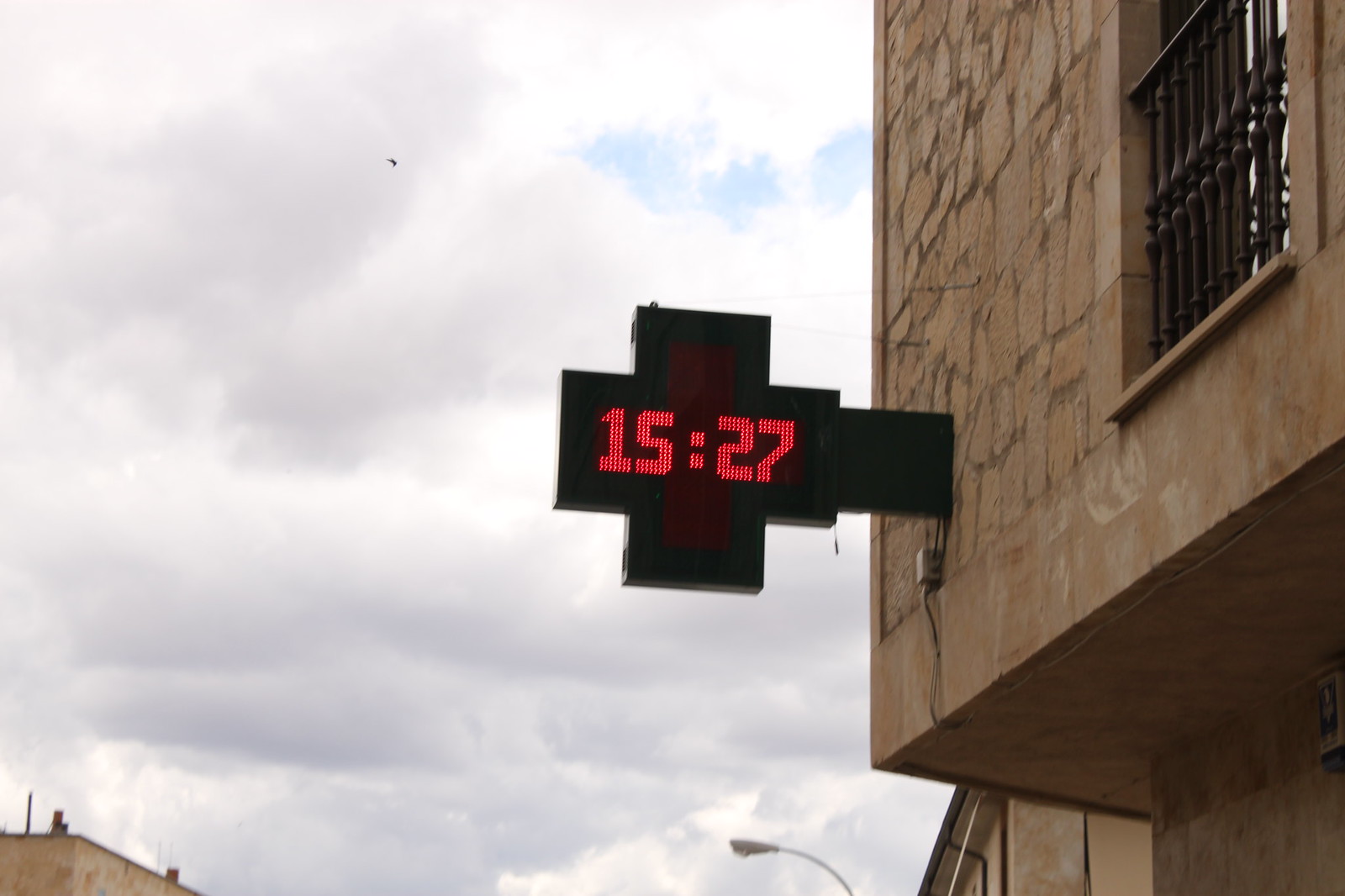This photograph captures the front of a brown brick building, prominently featuring a large, thick cross-shaped sign that appears to belong to a pharmacy or medical establishment. The sign displays the digital time "15:27," which is 3:27 in the afternoon. Adjacent to the sign, a dark brown, spindled balcony is visible on the building's second floor. The overcast sky is mostly gray with substantial cloud coverage, though patches of blue sky peek through in a few small areas. A streetlight can be seen in the frame, and another brown brick building is visible in the distant bottom left corner of the image. The photo appears to be taken from an elevated position, perhaps the second floor of a nearby building, offering a high vantage point.